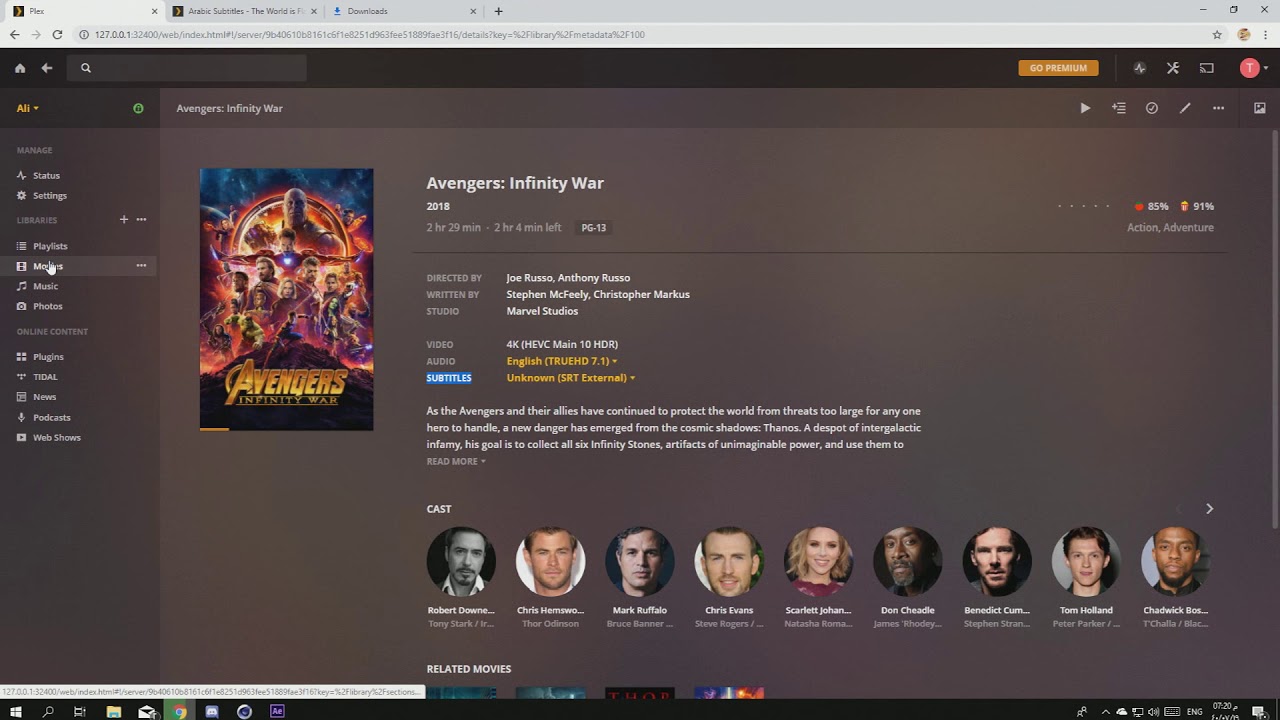A screenshot from a gaming interface displays detailed information about the movie **"Avengers: Infinity War" (2018)**. On the left side of the screen, there's an image representing the game. The movie is directed by **Joe Russo and Anthony Russo** and written by **Stephen McFeely**. Another credited individual is **Christopher Markus**. The film is produced by **Marvel Studios**.

The synopsis reads: 

"As the Avengers and their allies continue to protect the world from threats too significant for any one hero to handle, a new danger emerges from the cosmic shadows: Thanos, a despot of intergalactic infamy. His goal is to collect all six Infinity Stones, artifacts of unimaginable power..."

A "Read More" drop-down option is visible.

The cast list includes notable actors such as **Robert Downey Jr., Chris Hemsworth, Mark Ruffalo, Chris Evans, Scarlett Johansson**, and **Don Cheadle** among others. Below the movie information, there are related movies listed, though the details are partially cut off.